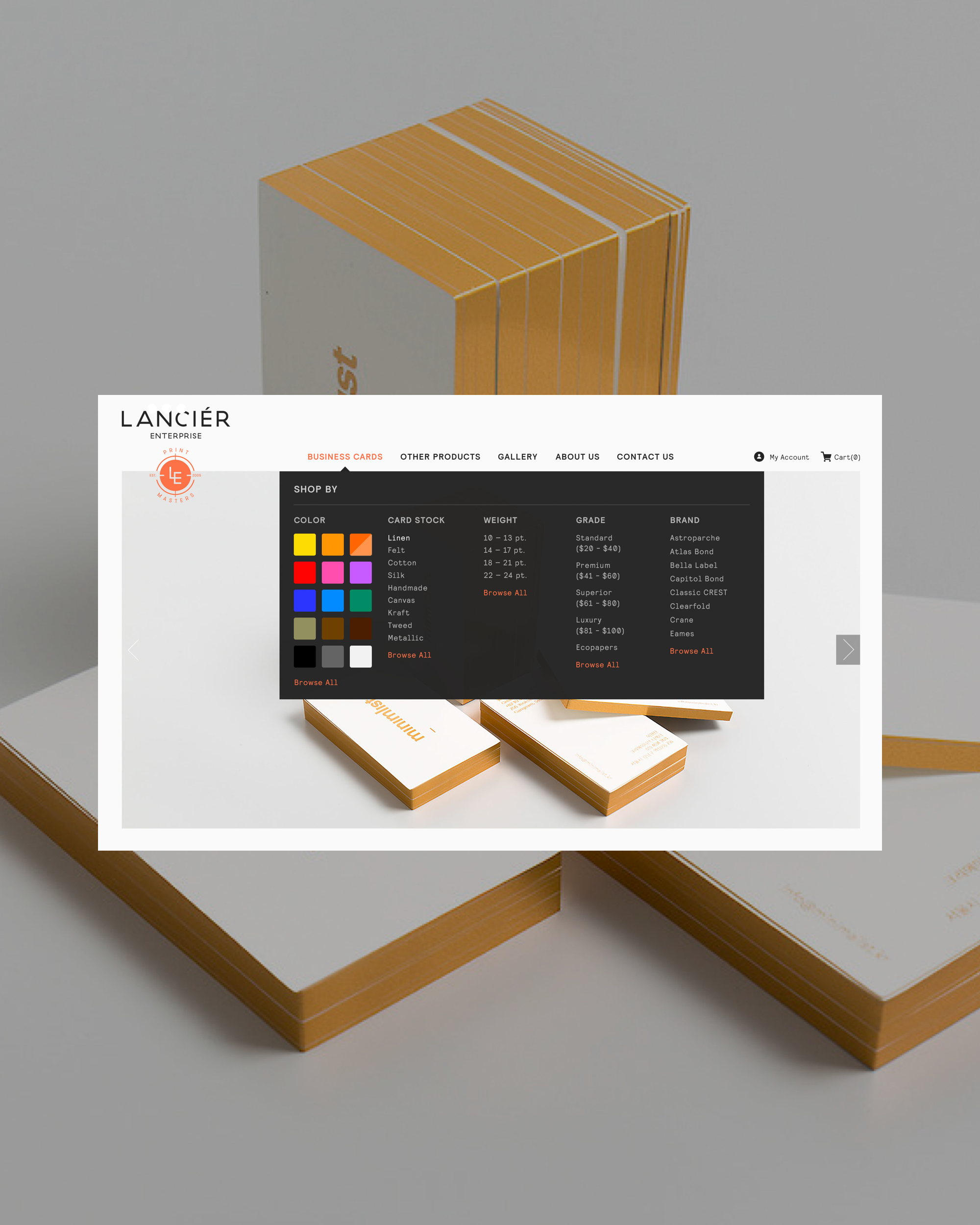This image appears to be a detailed screenshot taken from a website. The overall design is rectangular with a predominantly gray background. In the background of the image, there appears to be a photograph that resembles a collection of phone books or business card holders. These objects are white and stacked in various positions — two or three lying flat on a white table, and one large cube-shaped item standing upright. A few letters, including "S" and "T", are visible on this upright object.

Layered on top of this background image is a smaller horizontal rectangle located in the middle of the composition. This smaller image mirrors the background photograph but includes additional elements. In the upper left corner of this secondary rectangle, the text “Lancier Enterprise” is prominently displayed. Below this, a navigation menu includes options such as "Business Cards," "Other Products," "Gallery," "About Us," "Contact Us," "My Account," and "Cart."

Additionally, there is a small black pop-up box located above this secondary image, pointing towards the "Business Cards" section. To the left of this box, a color palette consisting of various colored squares is displayed, indicating customization options. The pop-up also lists different types of business card options, including "Card Stock," "Weight," "Grade," and "Brand." This indicates that the website allows users to create and personalize their own business cards by choosing various specifications.